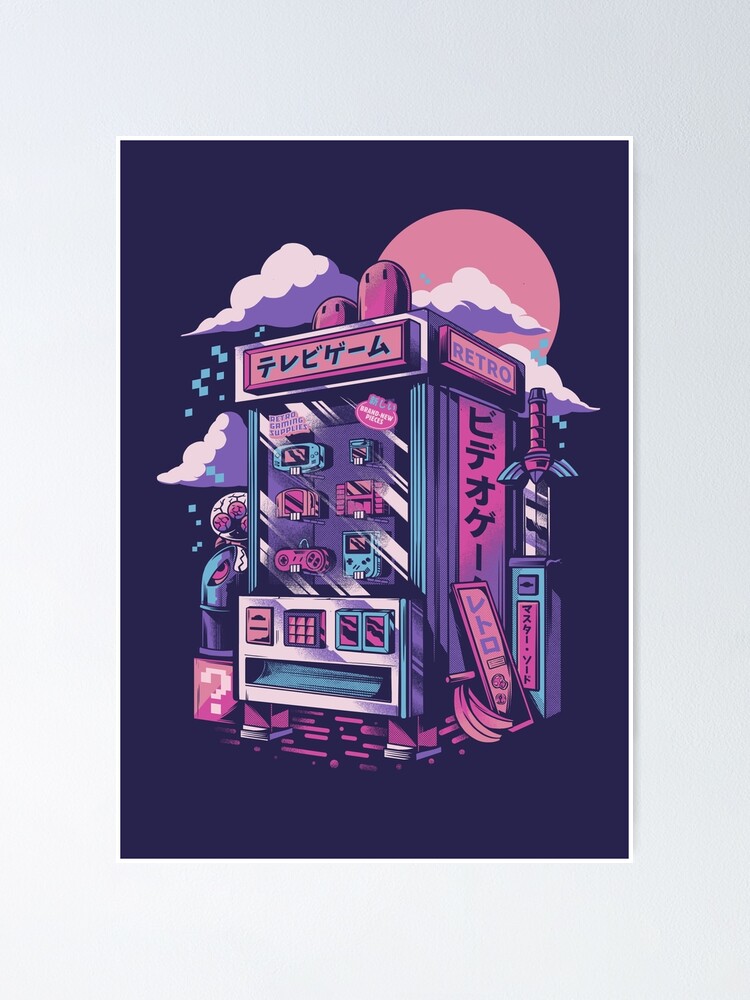This vertical, computer-generated artwork draws heavy inspiration from Japanese culture, featuring a vibrant, futuristic vending machine against a dark blue background. The vending machine is primarily adorned in shades of pink and purple, with intricate details highlighted by the contrasting dark backdrop. Accentuating the Japanese aesthetic, the machine showcases Japanese writing on the top and along the right-hand side.

Positioned towards the left, the vending machine is shown in a three-quarter view, revealing an array of nostalgic video game memorabilia behind its large window. Inside, you can spot a Super Nintendo controller, Game Boy, Game Boy Advance, Nintendo 64 games, and other retro gaming items. Below the window, there are multiple kiosk panels and a wide tray for dispensing items, alongside a silver-bordered slot.

At the top of the vending machine, two figures resembling Diglett from Pokémon and a black bullet, akin to those from the Super Mario series, enhance the thematic elements. A small box resembling a Super Mario question mark block with the bullet perched on top features prominently. On the right side, a sword with wings at the hilt extends vertically, flanked by Japanese signs and a couple of bananas at its base.

The background features a large, pink moon or sun partially obscured by whimsical clouds, which are white on top and gray underneath, further accentuating the artwork's fantastical and techie feel. Midway through the vending machine, the English word "Retro" is prominently displayed, reinforcing the nostalgic theme. Small blue pixels appear to rain down from the clouds, adding a dynamic and playful touch to the scene.